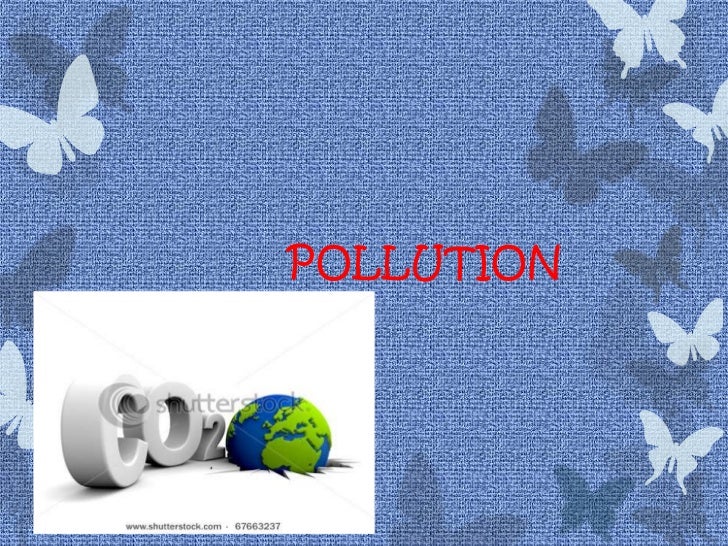The image features a textured blue background resembling denim fabric, with a visible weave pattern. Along the left and right edges are delicate silhouettes of butterflies in translucent white, through which the weave of the fabric is still discernible. These butterflies are accompanied by gray shadows, also translucent, adding depth to the visual. In the center, bold red capital letters spell out "POLLUTION." Positioned in the bottom left corner is a white rectangle containing large 3D letters reading "CO2," with a globe appearing to crash through the ground beneath the letters. Additionally, the corner includes text that reads "www.shutterstock.com 67663237." The entire image is overlaid with a Shutterstock watermark.